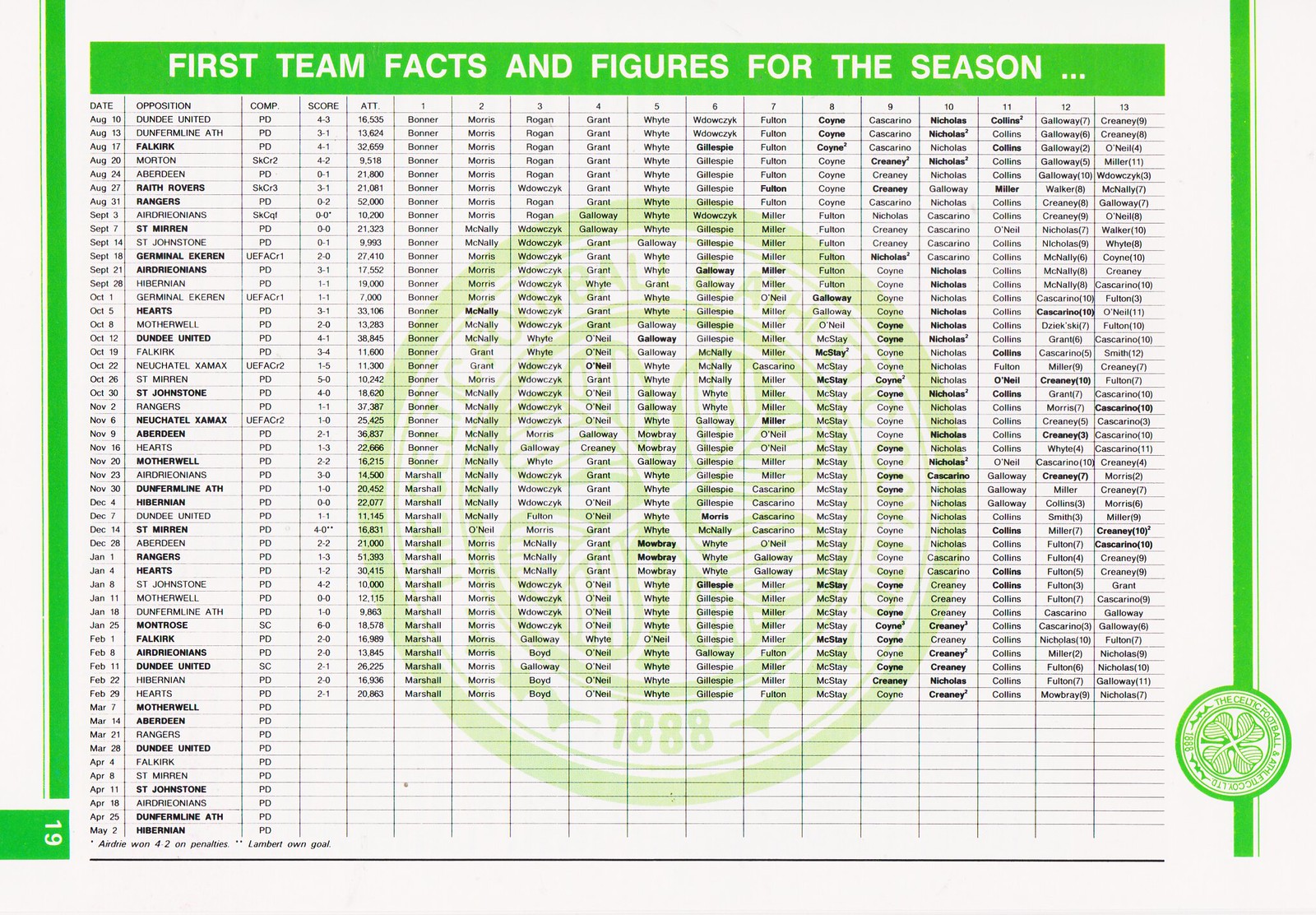The image depicts a highly detailed statistical chart predominantly in green and white, titled "FIRST TEAM FACTS AND FIGURES FOR THE SEASON" in bold white capital letters across a green banner at the top. The chart is structured into numerous columns, around 20 in total, each meticulously labeled. The rows, numbering between 50 to 100, are densely packed with data. On the far left, dates range from August to May, followed by columns labeled with headers such as "Comp," "Score," and "ATT," along with numbered columns from 1 through 13. Information under these labels includes player names and their respective game statistics. Centrally, a green circular emblem set against the white background features a four-leaf clover, symbolizing Celtic Football Athletic Limited, overlaying what appears to be a soccer ball. The small, dark print on the stat sheet details various aspects of the team's performance, from game dates and opponents to individual player achievements.